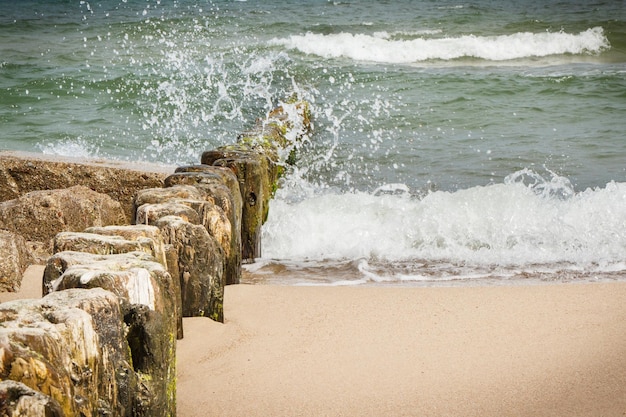In this vibrant daytime photo of a beach shore, a prominent wooden wave breaker extends vertically from the sandy beach into the ocean, standing out amid the crashing waves. Waves continually hit the shore, splattering white water against the weathered breaker and revealing successive waves rolling in. On the left side of the shore, there is a rock barrier composed of large, rectangular boulders that stretch into the water. These boulders, standing about two feet above the sand, are gray and dark brown with patches of green algae. The beach sand, a beige or peach color, occupies the lower right side of the image. The ocean has a striking dark green hue, with waves tumbling toward the shore and creating white foamy splashes upon impact. Further along the upper half and right upper corner of the image, additional waves can be seen crashing and forming white crests in the distance. The entire scene is filled with the dynamic energy of water splashing against the rocks, with droplets shooting upwards, and evokes a bright and lively coastal atmosphere.